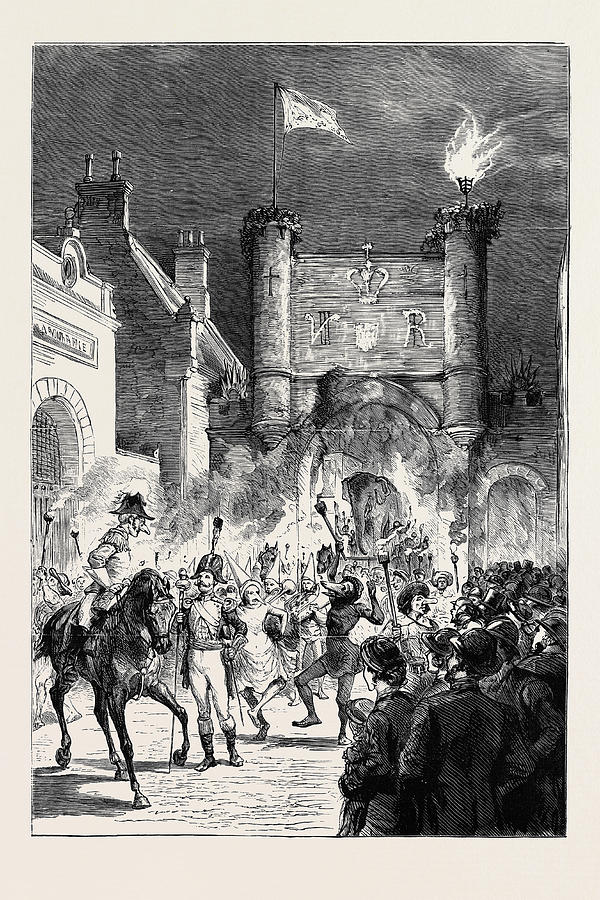The image is a detailed rectangular grayscale sketch measuring approximately 6 inches high and 3 inches wide, framed by an off-white border about a quarter inch wide on the sides and slightly wider at the top and bottom. Set against a backdrop of dark, intricately designed medieval or Renaissance-era architecture with towers, arches, and flags, the scene evokes a historical period from the 1500s to 1700s, perhaps even the French Revolutionary times.

In the foreground, a lively and curious crowd gathers, with men in top hats and bowler hats, women in Victorian dresses and sun hats, and a mother holding her child, both facing the viewer. Dominating the left side of the scene is an open field where a man on horseback, wearing a pointed hat with a feather and a plague doctor mask, looks down at another figure on the ground dressed in military attire. This soldier appears to be leading a parade with a staff in hand.

A significant portion of the crowd consists of people in costumes, featuring exaggerated long noses and pointed hats, reminiscent of plague-era disguises. Among them, a dancing man dressed as an animal waves his torch high in the air, and beside him, a woman in a white dunce cap dances, mirroring the playful and curious atmosphere. Torches are prevalent, adding a flickering light that contributes to the night-time setting of the sketch. The overall scene, full of detailed figures and dynamic action, appears to be some sort of festive parade or curious gathering, rich in historical and whimsical elements.